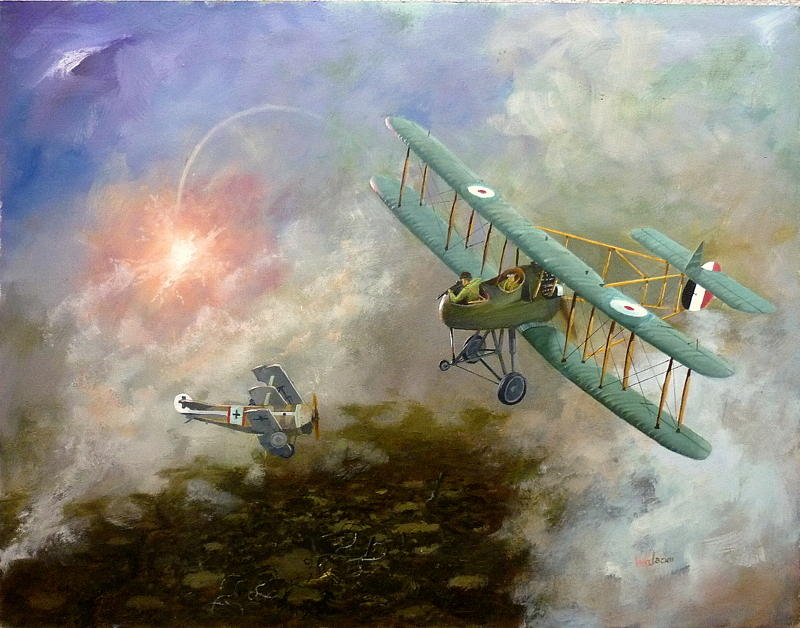This rectangular watercolor painting, approximately six inches wide by four inches high, vividly captures an aerial battle scene, possibly from World War II. The sky is artistically rendered with dramatic colors: a striking purple cloud mass on the left and smoky green hues on the right. The bottom left corner presents an explosion of pink and orange shades amidst smoky surroundings, suggesting a chaotic battle environment. 

In the sky, two military planes dominate the scene. The plane on the center-right, a blue glider-like aircraft with top and bottom wings connected by a brown metal frame, features two exposed pilots. The rudder at the back showcases vertical stripes of black, white, and red. The gunner is firing a black gun towards a white plane below. This white plane, adorned with three wings marked by white crosses and a propeller, is flying towards the right. It carries a banner featuring a red outer stripe, white center, and black equilateral cross. Above this plane is an explosion partly obscuring the sky.

The ground below is depicted in brown tones, while the overall setting encompasses various shades of blue, purple, white, green, tan, orange, brown, black, and gray. This intricate and expressive scene, devoid of any text, suggests it may be a hand-painted piece suitable for display in a museum.